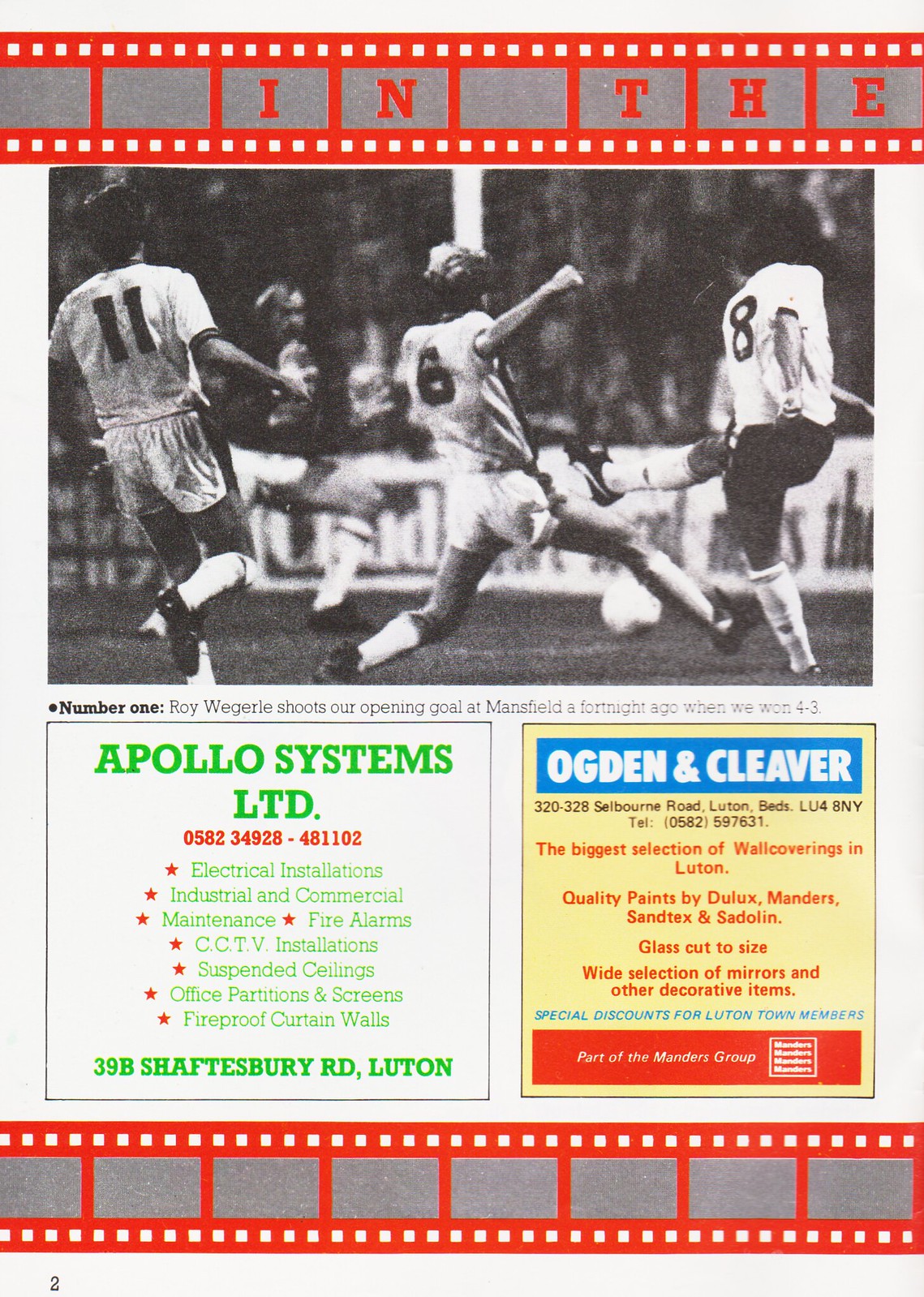This image is a color-printed page from a soccer club program, presented in portrait orientation. It features a prominent half-page black-and-white photograph of three soccer players in white jerseys, numbered 11, 6, and 8 from left to right, leaping into the air to play a ball. The players are seen in action against a backdrop of a packed stadium of spectators. Dominating the top and bottom of the page are banners designed to mimic a filmstrip, with an orange background, gray insets, and red text. The visible letters in the top banner spell out "NV," but the rest is cut off. Beneath the photograph, a caption reads: "Number one Roy Wegirl shoots our opening goal at Mansfield a fortnight ago when we won four to three.” Below this caption are two display ads from sponsors. On the left, an ad for Apollo Systems LTD is printed in green, listing services such as electrical installations, maintenance, and fire alarms, and includes a phone number in red. On the right, an ad for Ogden and Cleaver, set against a blue background, promotes the largest selection of wall coverings in Luton, with their address listed as Selborne Road, Luton. The overall style of the publication combines color printing with black-and-white photography to create a striking visual contrast.